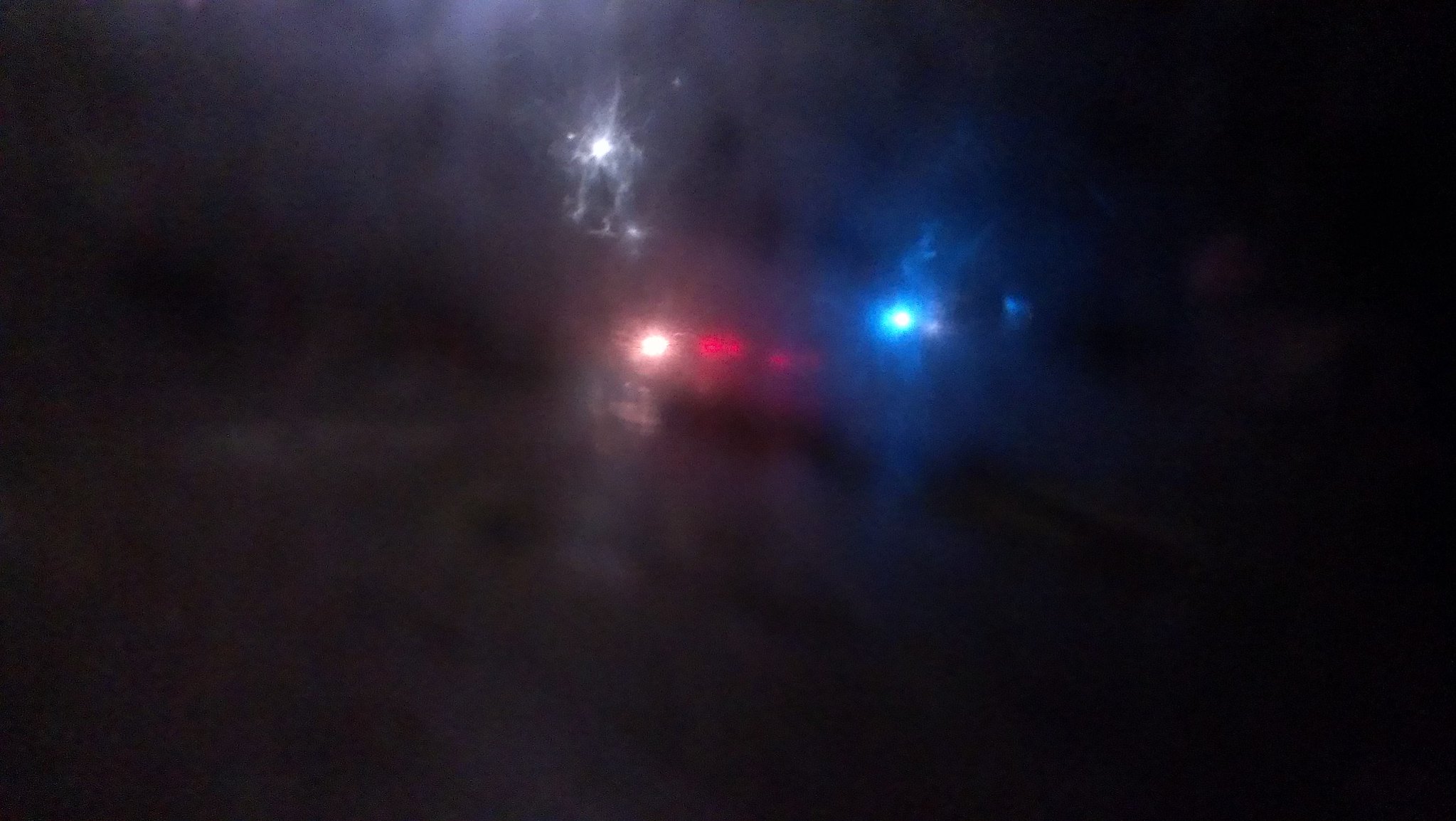The dark, nighttime photograph appears to be taken through a blurred, possibly foggy, windshield or obscured window, with a significant amount of grain or distortions. Dominating the scene are several indistinct lights: car brake lights glowing a faint red in the distance, a bright white street light hinting at oncoming traffic, and a vibrant blue light that stands out against the nighttime backdrop. The overall image is heavily blurred, skewed, and doubled, likely due to the foggy conditions and the motion of the car. Amidst this spectral setup, an illuminated full moon hangs in the sky, casting a faint glow on the surrounding clouds, further enhancing the ethereal and enigmatic atmosphere of the photograph.